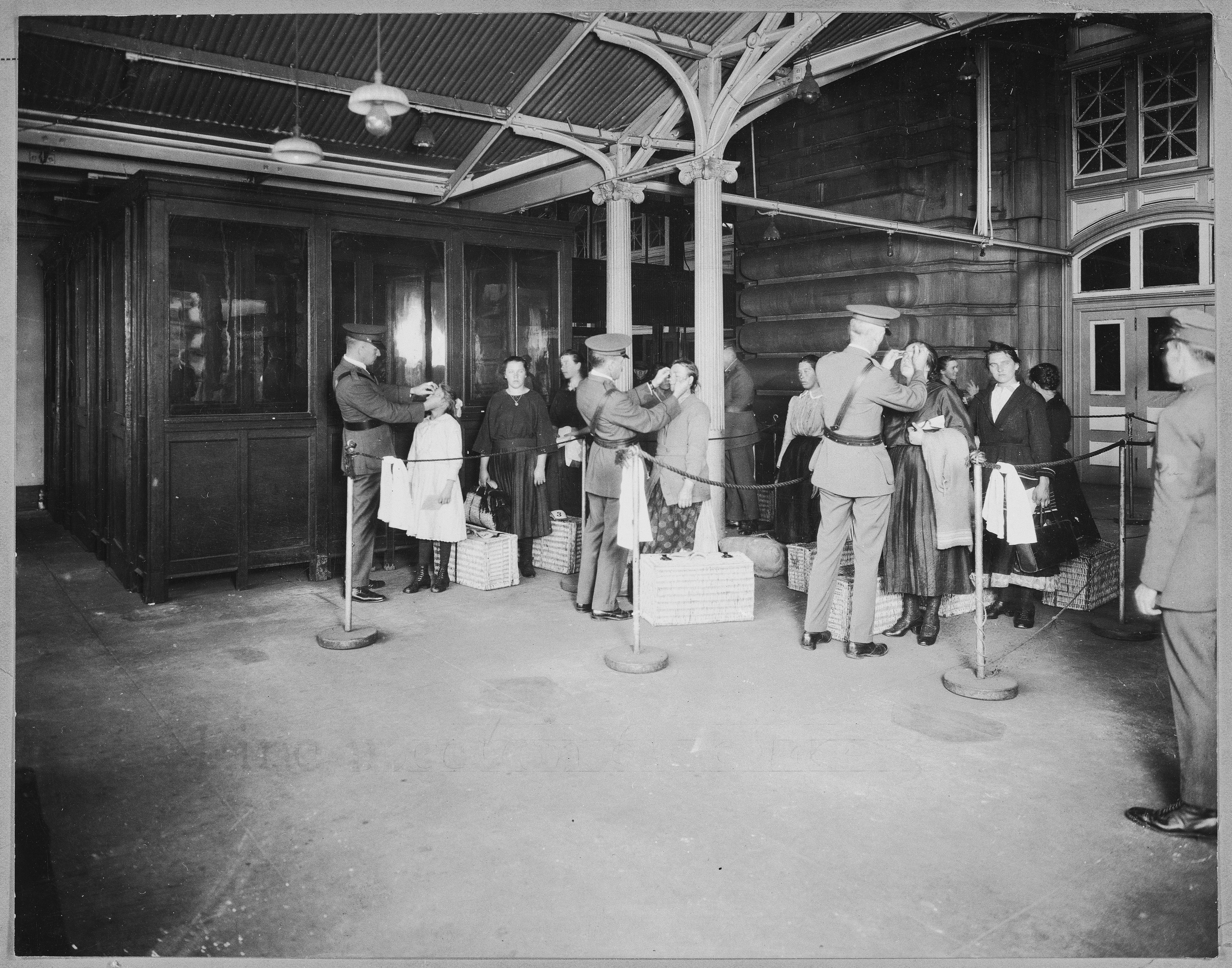This vintage black-and-white photo captures a scene likely set in the 1920s, 30s, or 40s, inside a train station with a ticketing booth or office area visible in the background. The photo is filled with an air of tension and orderliness, as women dressed in old-fashioned clothing, complete with stockings and boots, stand in three roped-off lines. Each woman clutches a large basket or suitcase and wears a serious expression, suggesting a significant and potentially stressful moment, possibly immigrating or undergoing an inspection.

Five soldiers in formal uniforms oversee the process. Three soldiers, positioned in front of each line, appear to be inspecting the women's faces closely, almost as if looking into their eyes. Another soldier stands to the right, vigilantly watching the proceedings. Above, scaffolding with hanging lights illuminates the concrete floor. The orderly arrangement of people and the soldiers' meticulous attention indicate a controlled and systematic operation, set against a backdrop that hints at both the mundane and the momentous.